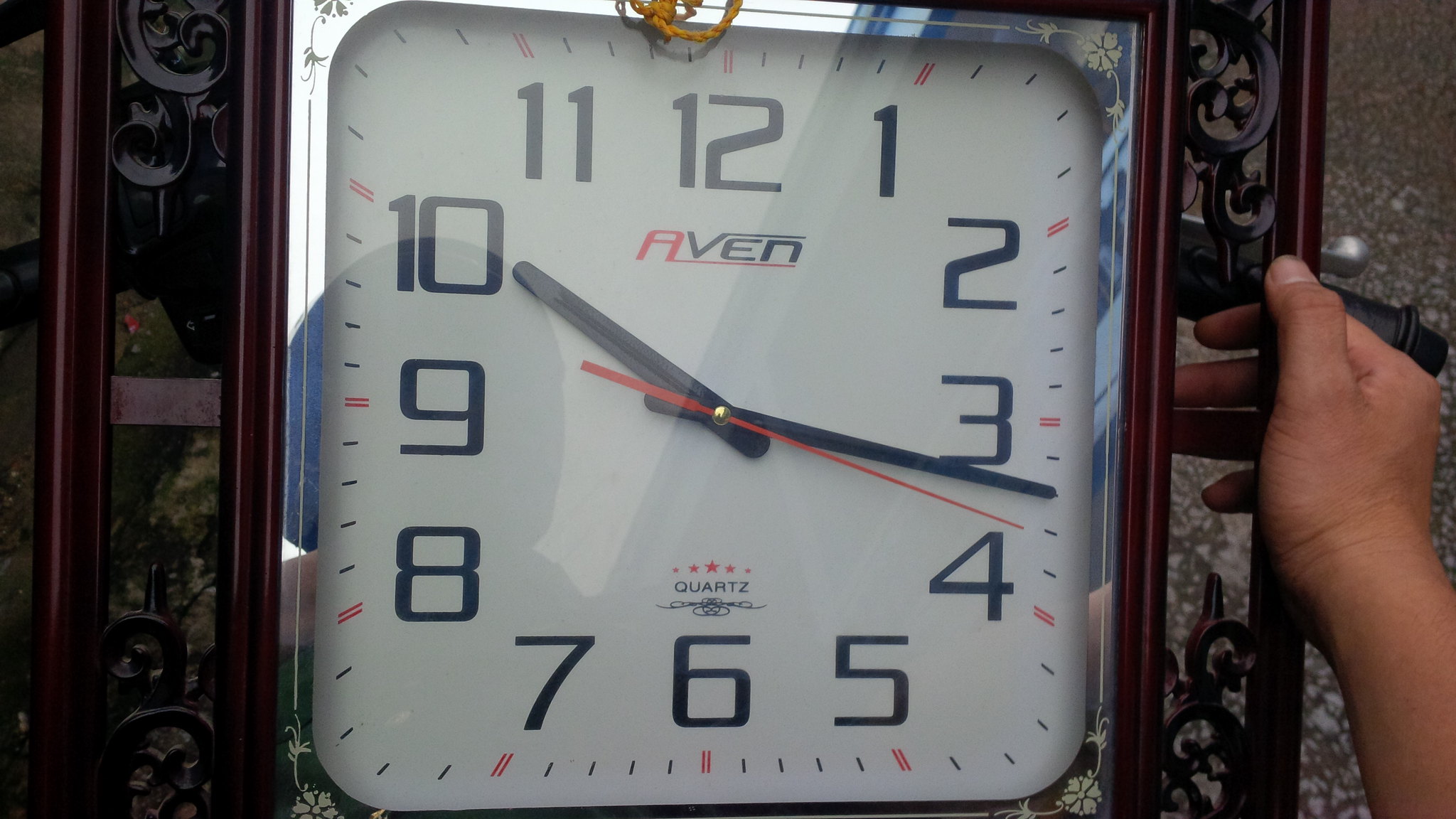This photograph features a square wall clock with a minimalist white face and bold black numbers ranging from 1 to 12. The clock's design includes black minute and hour hands, sharpening the contrast against its white background. A vibrant red second hand adds a touch of color and dynamism to the composition. The clock displays the time as 10:17.

The clock face prominently features the brand name "FIVER" just below the number 12, cleverly styled with a color scheme that distinguishes each letter. The letters "F" and "I" are in vibrant red, while the remaining letters "V", "E", and "R" are in black. Notably, the "V", "E", and "N" are intertwined with the digit "5", adding a unique and artistic flair to the design.

A brown-skinned hand is seen holding the clock up on the right side, indicating a sense of human interaction with the object. This detail adds a personal touch to the otherwise ordinary timepiece, making the image more dynamic and engaging.